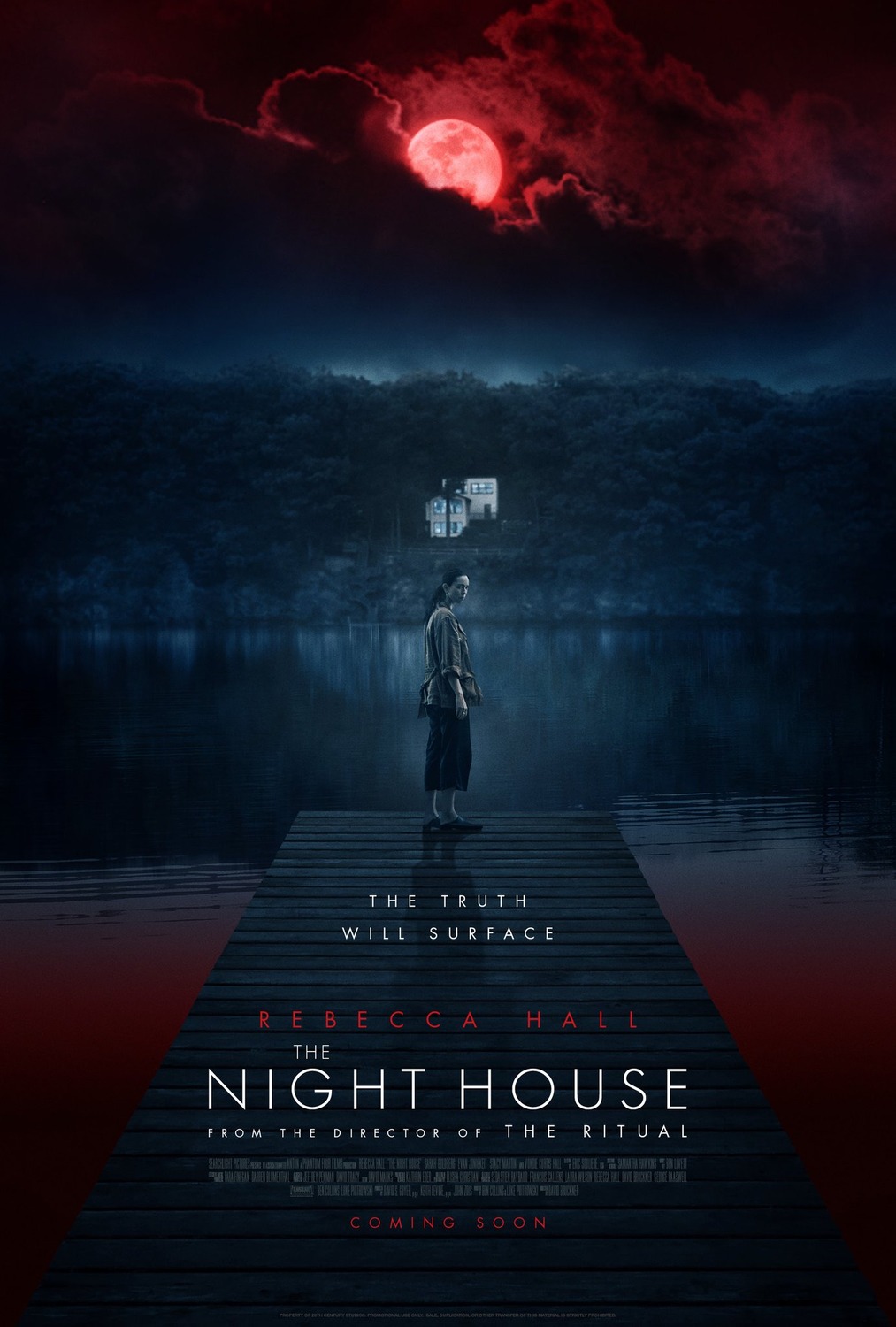This is a movie poster for "The Night House," featuring actress Rebecca Hall. The poster depicts a young woman standing at the end of a blackish-gray wooden pier that extends into a dark, ominous lake with swirling black, gray, and white hues. The woman, whose long black hair is tied back in a ponytail, is wearing knee-length black shorts, black shoes, and an untucked brown blouse. She stands facing to the right, slightly turned toward the viewer, in a contemplative pose. 

In the background, on the far shore of the lake, there is a two-story white house nestled amidst a dense line of dark trees. The house stands illuminated by a reflection from the moon. The sky overhead is a midnight blue with scattered clouds and features a partially visible, strikingly red moon speckled with small dots. Above the scene, in large white text, it reads: "The Truth Will Surface." Below that, in larger white text, is the movie's title, "The Night House," accompanied by the annotation, "From the Director of The Ritual." At the bottom, in red text, it announces: "Rebecca Hall," and "Coming Soon."